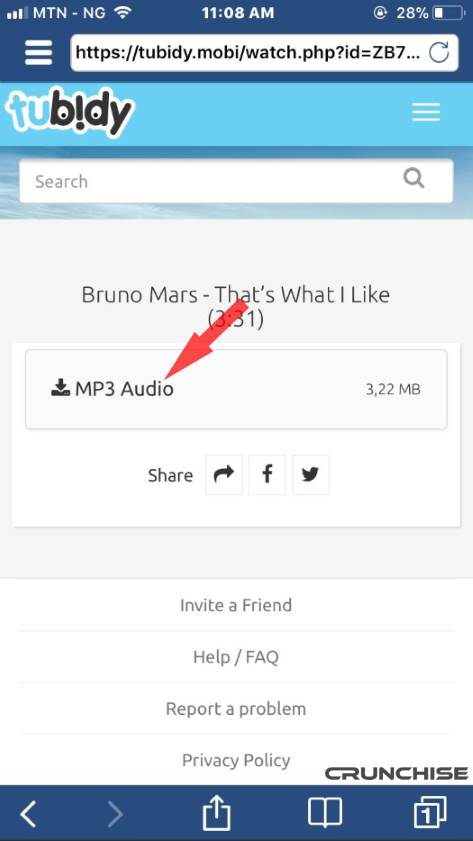The image depicts a smartphone screen displaying a website, specifically "Tubidy.mobi," a popular platform for downloading media files. 

The top of the screen features a blue header with essential status indicators: three horizontal bars representing signal strength, the text "MTN-NG" indicating the network provider, a Wi-Fi icon, the time displayed as 11:08 AM, a lock icon suggesting a secured connection, and a battery meter indicating 28% remaining charge. Below this header on the left, a hamburger menu icon is present.

The URL bar shows the website address "https://tubidy.mobi/watch.php?id=zb7..." and below this is the Tubidy logo. The logo integrates light blue and black text, with unique design elements: the letters 'T' and 'U' are colored in light blue, the 'B' and 'D' have dots embedded in them, and an inverted 'I' forms a face with a surprised expression, all set against a light blue background. Another hamburger menu icon sits on the right side of the header.

Beneath the header and logo, there’s a search field set against a sky background, currently empty. Search results are displayed below this field, starting with a listing for "Bruno Mars - That's What I Like," which has a duration of 3 minutes and 31 seconds. The file is available as an MP3 audio download, showing a file size of 3.22 MB. A distinct red arrow points to the word “audio” in the listing.

Further down, there are options for sharing on Facebook and Twitter, as well as additional functionalities like inviting a friend, seeking help, reporting a problem, and reviewing the privacy policy. The bottom of the site features a logo for "Crunchice" and a navigation menu with directional options (forward, backward, and upward). Additionally, there's a pagination control with a box displaying the number "1."